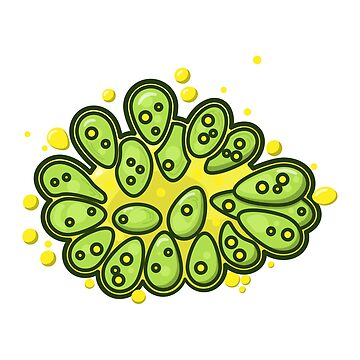The image is a cartoon-like illustration of an oleaginous green microalgae, set against a white background. The central focus is a yellow mass with globules of yellow substance dispersed around it, possibly representing lipid particles. Within this yellow mass, there are approximately 20 teardrop or oval-shaped green algae structures, some appearing somewhat egg-like. Each green structure is bordered by a thick black outline and contains smaller circles or dots, numbering between two to three, which are also yellow and have thick black borders. The green algae clusters are arranged elliptically around the central yellow mass, adding to the intricate, detailed depiction of the microalgae. This illustration, designed with a sticker-like style, vividly portrays the components and arrangement of the algae, although the exact scientific context remains ambiguous.